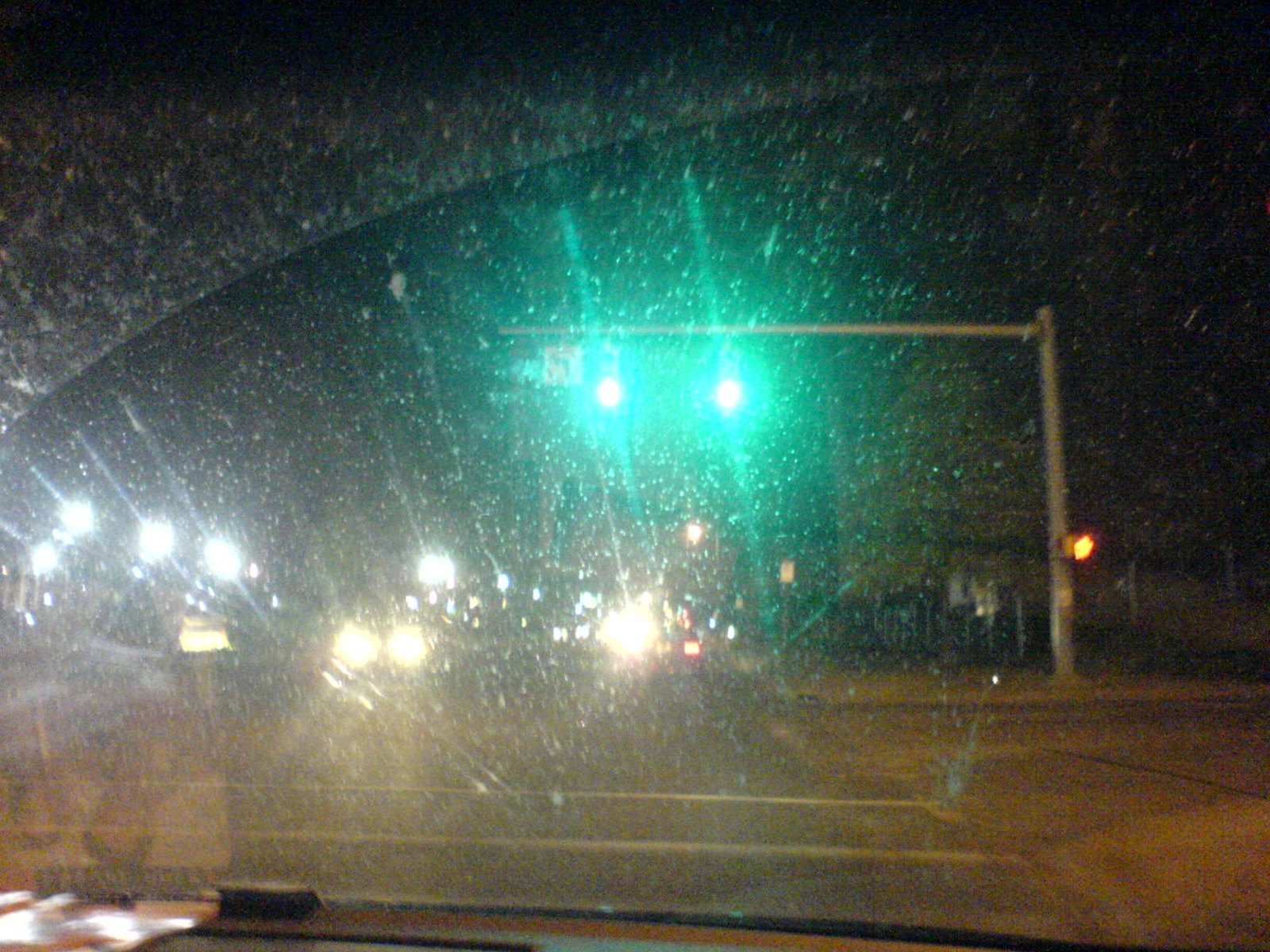The image captures the view through the windshield of a vehicle, which is noticeably dirty with numerous speckles, likely from rain or dirt, making visibility quite poor. The vehicle is crossing an intersection under a green traffic light, just beyond the crosswalk. On the opposite side of the intersection, there are at least two or three vehicles approaching, their outlines somewhat blurred due to the dirty windshield and poor visibility. A pair of bright white streetlights can be seen on the left-hand middle side of the photo. Towards the center, two or three vehicles are more discernible. In front of the photographing vehicle, red tail lights from another car are visible, slightly beyond the intersection. The traffic lights above the intersection are mounted on a gray horizontal bar and both show green, indicating it is safe to proceed. The pedestrian crosswalk signal shows "Don't Walk," suggesting it may soon change. The overall scene is one of cautious movement through the intersection amidst the challenging visibility conditions.